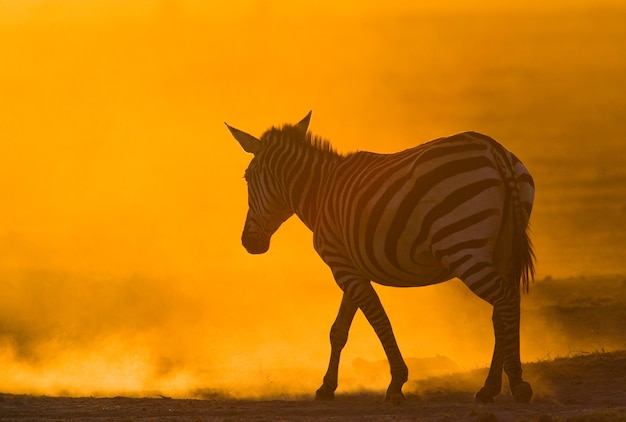In the distance, a zebra with classic black and white stripes is seen through a hazy, orange-tinted atmosphere. The zebra, characterized by its small ears and thin, wispy mane resembling a short mohawk, has a drooping tail with a bit of hair at the end. It is slowly walking away from the viewer towards the left. The setting sun casts a golden hue on the surrounding dust clouds, creating a smoky, orange glow that envelops the scene. The dry, arid ground is dotted with small patches of brown grass, further emphasizing the desolate, desert-like environment.